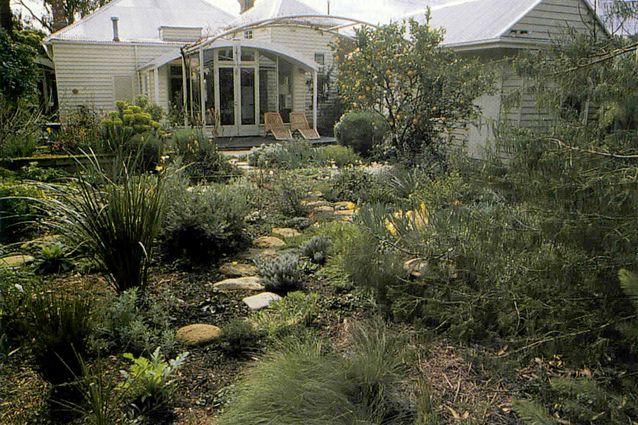An image captures what seems to be the backyard of a house with a beigeish color and lateral shingles. The space is lush with greenery, exhibiting an impressive biodiversity including several bushes, smaller plants, and trees, one of which might be a lemon tree. Wild grass and weeds freely grow, adding to the feeling of an overgrown, somewhat abandoned garden. There is an aged cobblestone path, made from large stones, curving gently towards a set of glass French doors on the house. A patio area, possibly once covered but now partially broken, features two beige wicker chaise lounges. The backyard is rich with various plant life and conveys a sense of natural, untamed beauty, despite the apparent neglect of both the house and its surroundings. To the right, there appears to be an additional structure with white siding and a white pitched roof, possibly a shed or another small building. Overall, it's a humble abode with a verdant, slightly wild character.